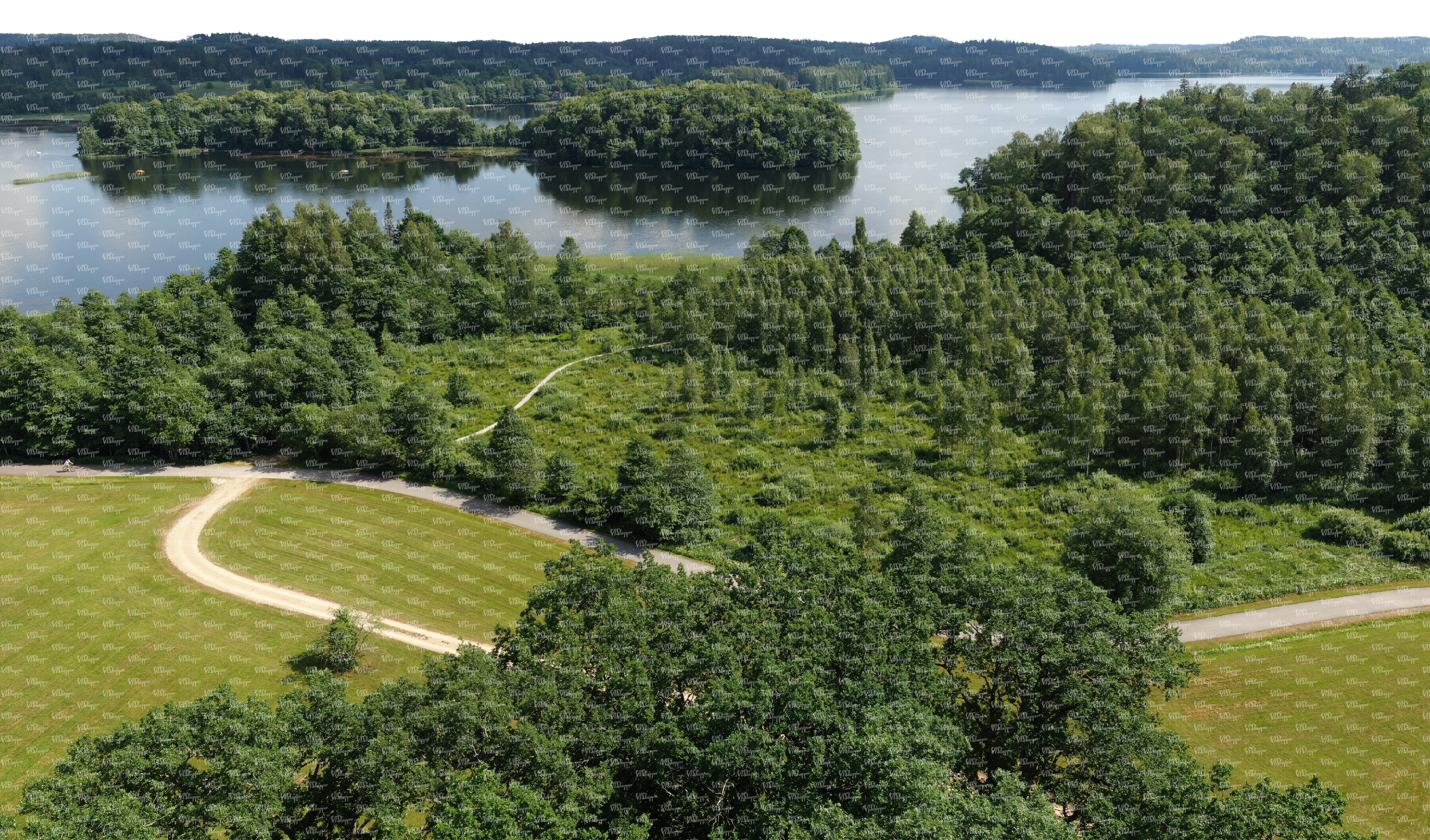The aerial photograph captures a stunning, sunlit landscape featuring a long, winding road meandering through a flat, grassy expanse. In the middle and to the left of the image, the road zigzags before continuing out of view, flanked by small dirt paths. Surrounding this grassy area is a dense forest that extends towards a wide, grayish river. Scattered across the river are tree-covered islands, with more forested land visible beyond the water. The scene is framed by small hills and a bright, clear sky, providing a picturesque bird's-eye view of the verdant environment. Along the grassy expanse, countless tiny water marks add subtle texture to the overall panoramic scenery.